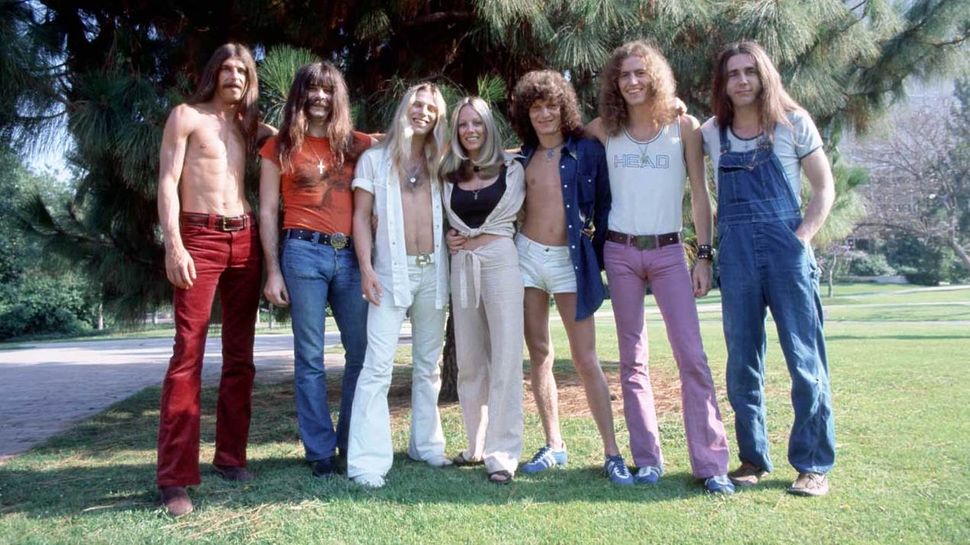In this sharp and vibrant photograph, likely taken during the 1970s or 1980s, seven individuals stand side-by-side, posing serenely in front of a large, leafy tree. The clear image captures the essence of a sunny day, with each person casting distinct shadows on the lush, green grass beneath them. A small house peeks out from the background to the right, and a winding road encircles the scene, adding depth to the picturesque setting.

Among the seven, six are men and one is a woman who stands prominently in the center. The woman sports blonde hair parted in the middle and is dressed in beige pants, a black shirt, layered with a white overshirt. Her companions, sporting long hair of varying shades and textures—brown, blonde, straight, and curly—appear equally relaxed and carefree. One man stands out in short white shorts, while the rest wear jeans, with the exception of one in overalls, adding a casual and nostalgic flair.

Several of the men are partially bare-chested; one without a shirt altogether, and two with open shirts revealing their chests. The casual 70s/80s style is further accentuated by their accessories, as most are adorned with necklaces. All seven individuals are smiling warmly, exuding a sense of camaraderie and joy as they bask in the sunlit moment captured perfectly by the camera.